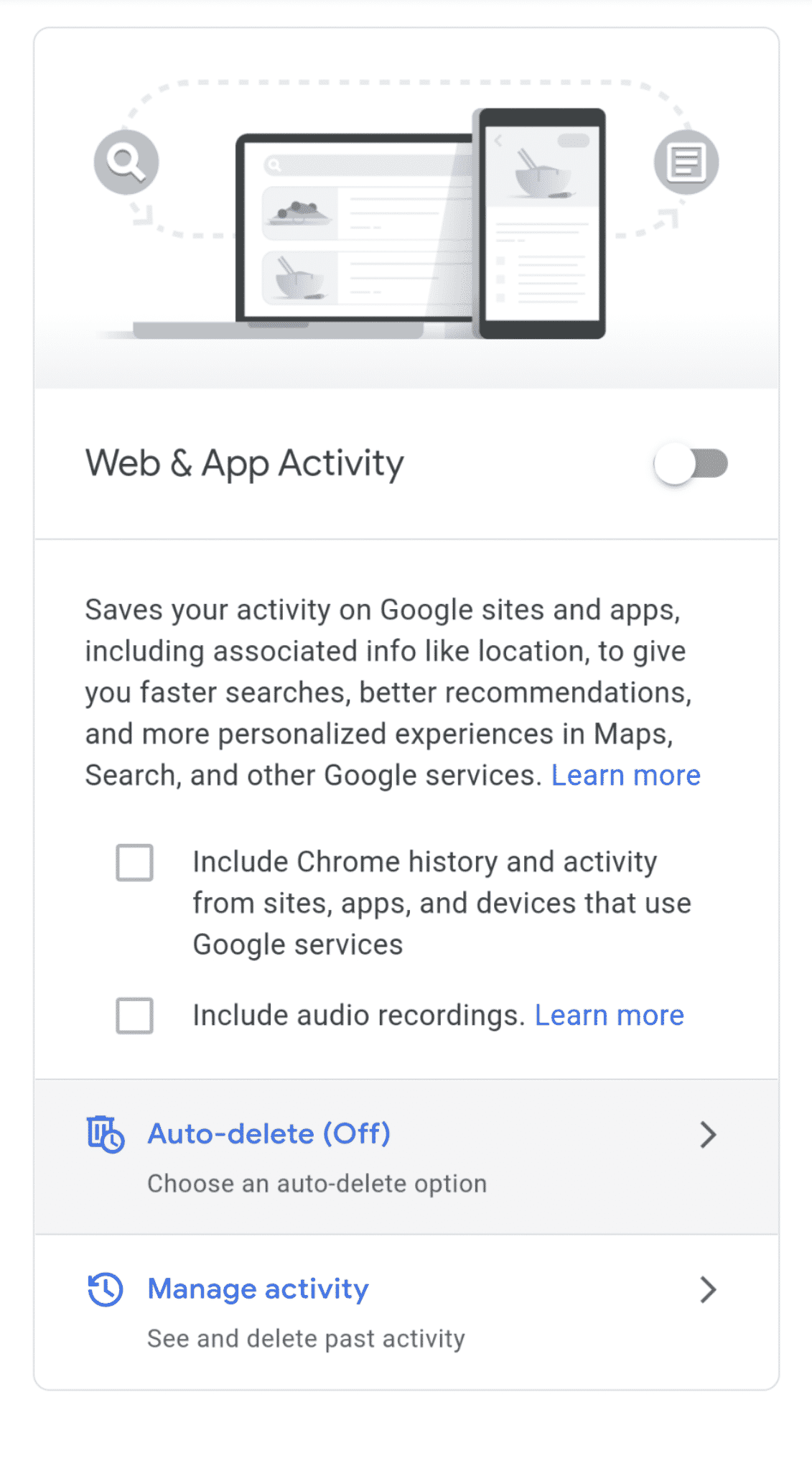The image is a screenshot of the settings section of a website, showcasing a grayscale, cartoon-like illustration at the top. This illustration depicts a laptop with a smartphone positioned to its right. Beneath this image, the text reads "Web & App Activity," with a toggle switch that appears to be turned off. The description below the toggle explains that enabling this setting saves your activity on Google sites and apps, including associated information like location, to provide faster searches, better recommendations, and more personalized experiences in services such as Maps and Search.

Additionally, there are options to include Chrome history and activity from sites, apps, and devices that use Google services, with an unchecked box next to this option. Another unchecked box allows the inclusion of audio recordings. Further down, the settings indicate that auto-delete is turned off, with an option to choose an auto-delete preference. At the bottom, there is a "Manage Activity" link, which allows users to see and delete past activities, accompanied by a right-pointing arrow at the end of the text.